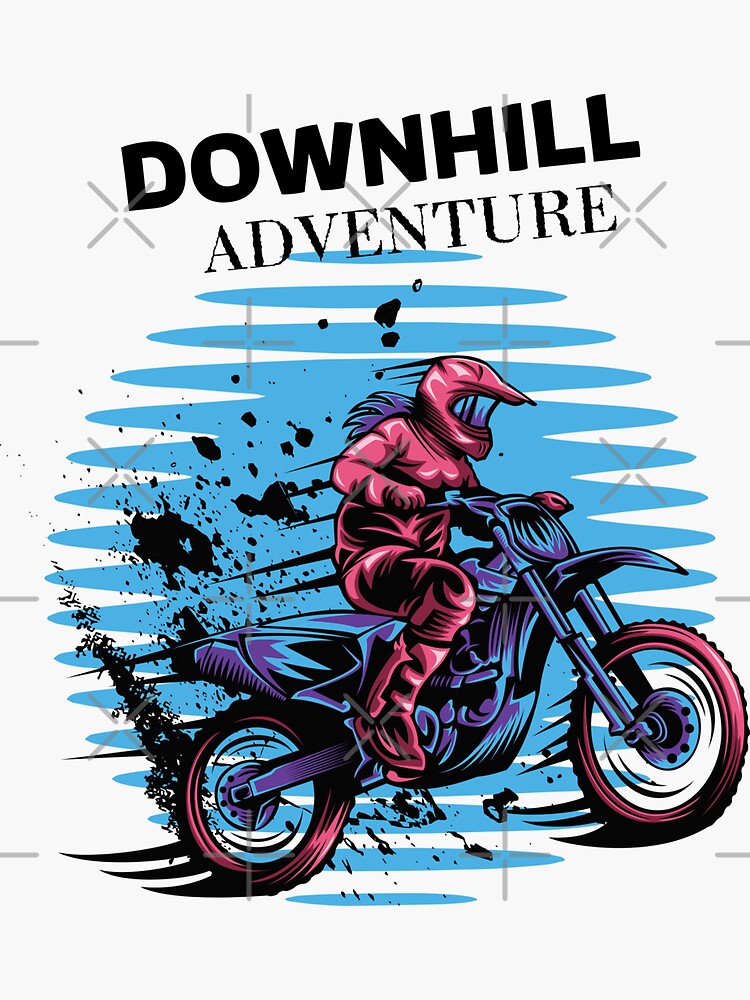The image appears to be a dynamic, action-packed book cover titled "Downhill Adventure." Set against a gray background, the title text is boldly angled in black, with "Downhill" in a thicker font and "Adventure" appearing in a more delicate, thin style. The cover features a prominent figure, likely a woman, illustrated or painted in vibrant colors. She is clad in a striking red outfit with black inlays, including matching boots, and sports a helmet with reflective glasses. Her long hair flows down her shoulder, reinforcing the impression that the rider is female. She speeds on a large, purple and teal motorcycle with pink wheels, exuding a sense of adventure and thrill. The image is artistically enriched with black ink blot splotches scattered across the center, and the backdrop includes a circle reminiscent of the AT&T logo, filled with interspaced blue and white lines. Additional details suggest the presence of watermarks in the form of X's and plus signs, indicating the artwork is copyrighted. The entire scene is drawn with markers and black pen, emphasizing the action and excitement central to the book's theme.